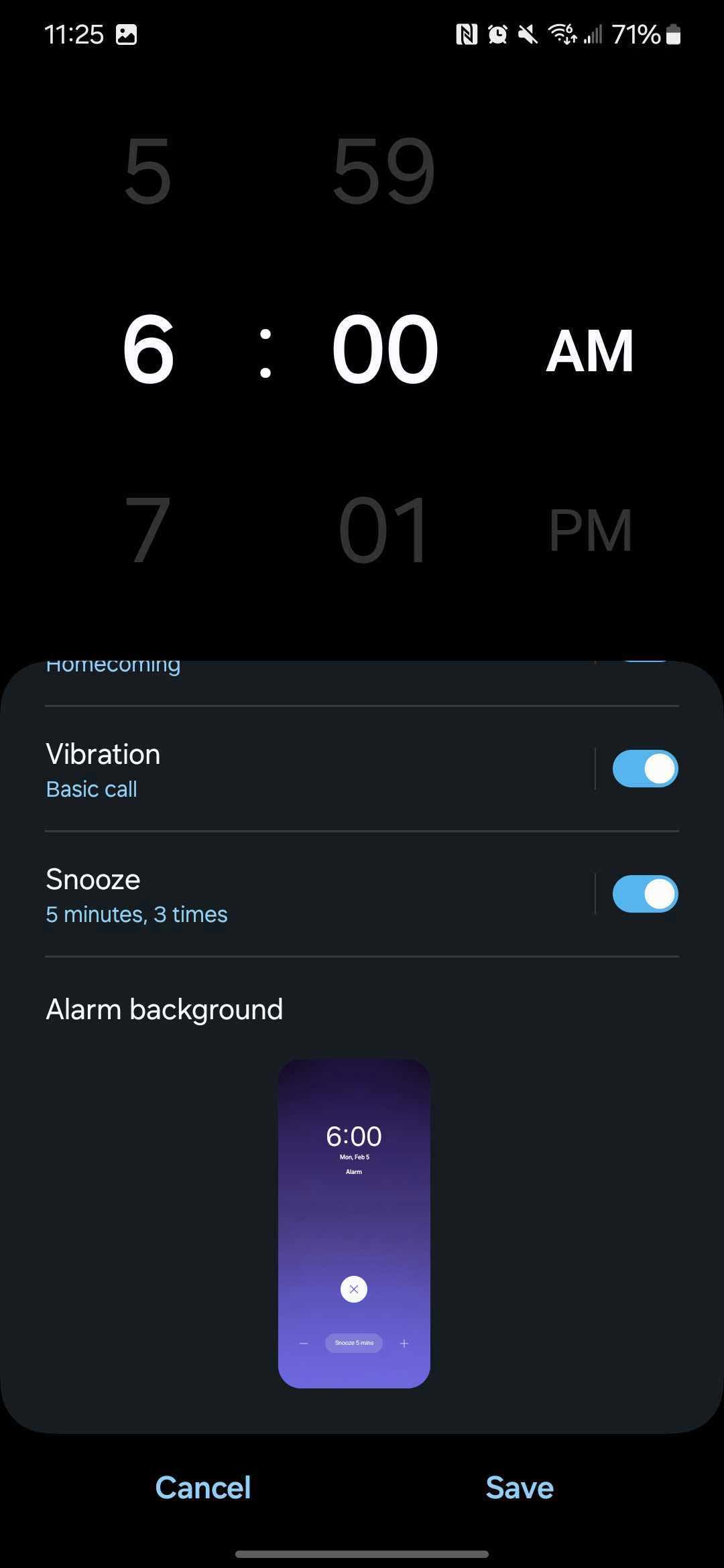The image depicts a smartphone screen with a predominantly black background, likely a screenshot of an alarm setting interface. The phone's status bar at the top shows the time as 11:25 AM and indicates the battery level at 71%. Below the status bar, there is a large digital clock displaying "6:00 AM" in bold digits, signaling the set alarm time. Above the main alarm time, "5:59" appears grayed out, indicating the approaching minute, and below, "7:01 PM" is also grayed out, possibly denoting another set time or the time after a snooze.

Beneath the clock display, a section outlines the alarm's configuration details. It lists "Vibration" and "Basic call" under alarm sound settings, both of which are turned on. The snooze functionality is activated with a setting of five-minute intervals, allowing up to three repetitions. Following this is the "Alarm background" section, where a preview image shows the phone's alarm screen with a simple blue backdrop.

At the bottom of the screen on a black background, two buttons are presented: "Cancel" in blue on the left and "Save" in blue on the right, offering options to either discard or save the alarm settings.